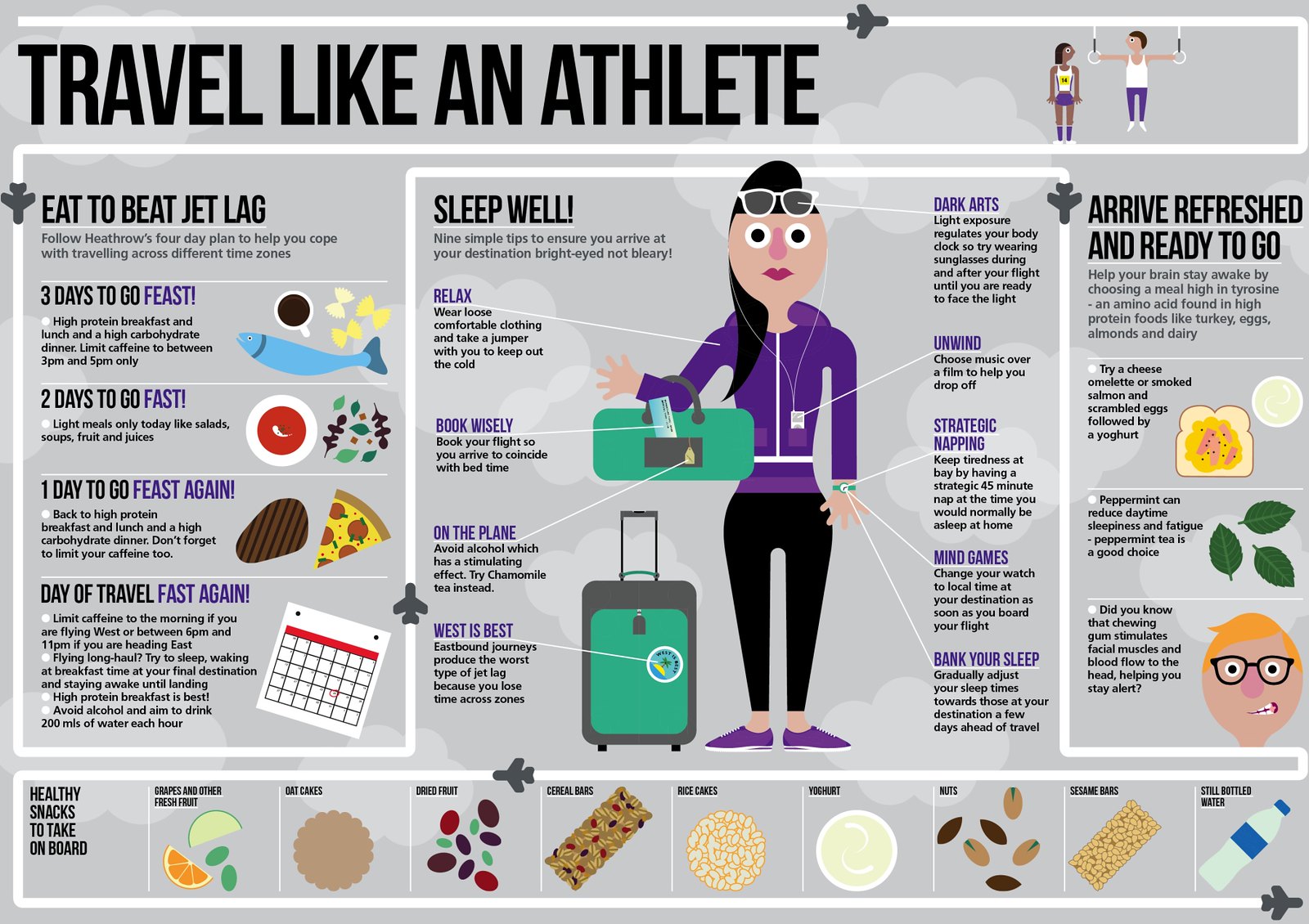The image depicts a detailed and colorful pamphlet titled "Travel Like an Athlete." The central figure is a cartoon drawing of a young woman wearing a purple jacket, black leggings, and purple shoes, carrying luggage and a purse. To the left of this central figure, there's a detailed chart themed around beating jet lag, labelled "Eat to Beat Jet Lag." It outlines a four-day dietary plan designed to help travelers cope with time zone changes, illustrated with cute drawings: 

- Three days before travel, "feast" on foods like fish, pasta, and coffee.
- Two days before, "fast" with lighter meals, including soup.
- One day before, "feast" again with hearty foods like steak and pizza.
- On the day of travel, "fast" again.

Adjacent to this, the pamphlet advises, "Sleep well, relax, and book wisely" while emphasizing that westbound journeys are preferable as eastbound causes worse jet lag. Additional travel tips are presented under catchphrases like "Dark Arts," suggesting controlled light exposure by wearing sunglasses, and "Unwind," recommending listening to music over watching films to fall asleep. "Strategic Napping" highlights the importance of 45-minute naps aligned with your home time zone, and "Mind Games" suggests changing your watch to local time upon boarding. 

On the right side, under the heading "Arrive Refreshed and Ready to Go," it discusses activities and preparations to help you feel rejuvenated upon arrival. This section includes images of an omelet and cheese sandwich, and a peppermint leaf, and mentions that chewing gum can stimulate facial muscles and blood flow.

At the bottom, another box lists "Healthy Snacks to Take on Board," featuring illustrations of grapes and other fresh fruits, oatcakes, dried fruit, granola bars, rice cakes, yogurt, nuts, sesame bars, and still bottled water. 

Overall, the pamphlet, possibly provided by Heathrow, is packed with comprehensive, illustrated advice for travelers looking to optimize their trips and arrive in peak condition.